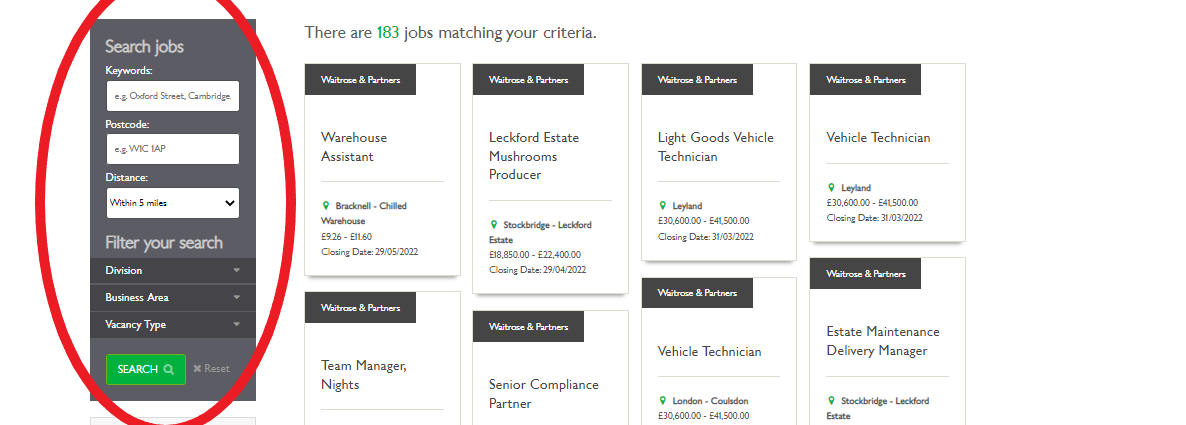The image depicts a section of a job search website interface, specifically a search function located on the left-hand side. Users can filter job listings by entering keywords, specifying a postal code (or zip code), and setting a preferred distance range. Below these fields, a green "Search" button allows users to execute the search.

A prominent thick red circle highlights the search box area. Adjacent to this, the interface indicates that there are 183 jobs matching the current search criteria. Job listings are displayed in a vertical column, each separated into distinct boxes with black-and-white designs.

The visible job titles include:
- Warehouse Assistant
- Lackford Estate Mushrooms Producer
- Light Goods Vehicle Technician
- Vehicle Technician
- Team Manager (Nights)
- Senior Compliance Partner
- Vehicle Technician
- Estate Maintenance Delivery Manager

Each listing provides a brief overview including the job title, an approximate salary range, and a closing date for applications. However, the lower section of the list is partially obscured, showing only the job titles of the remaining positions.